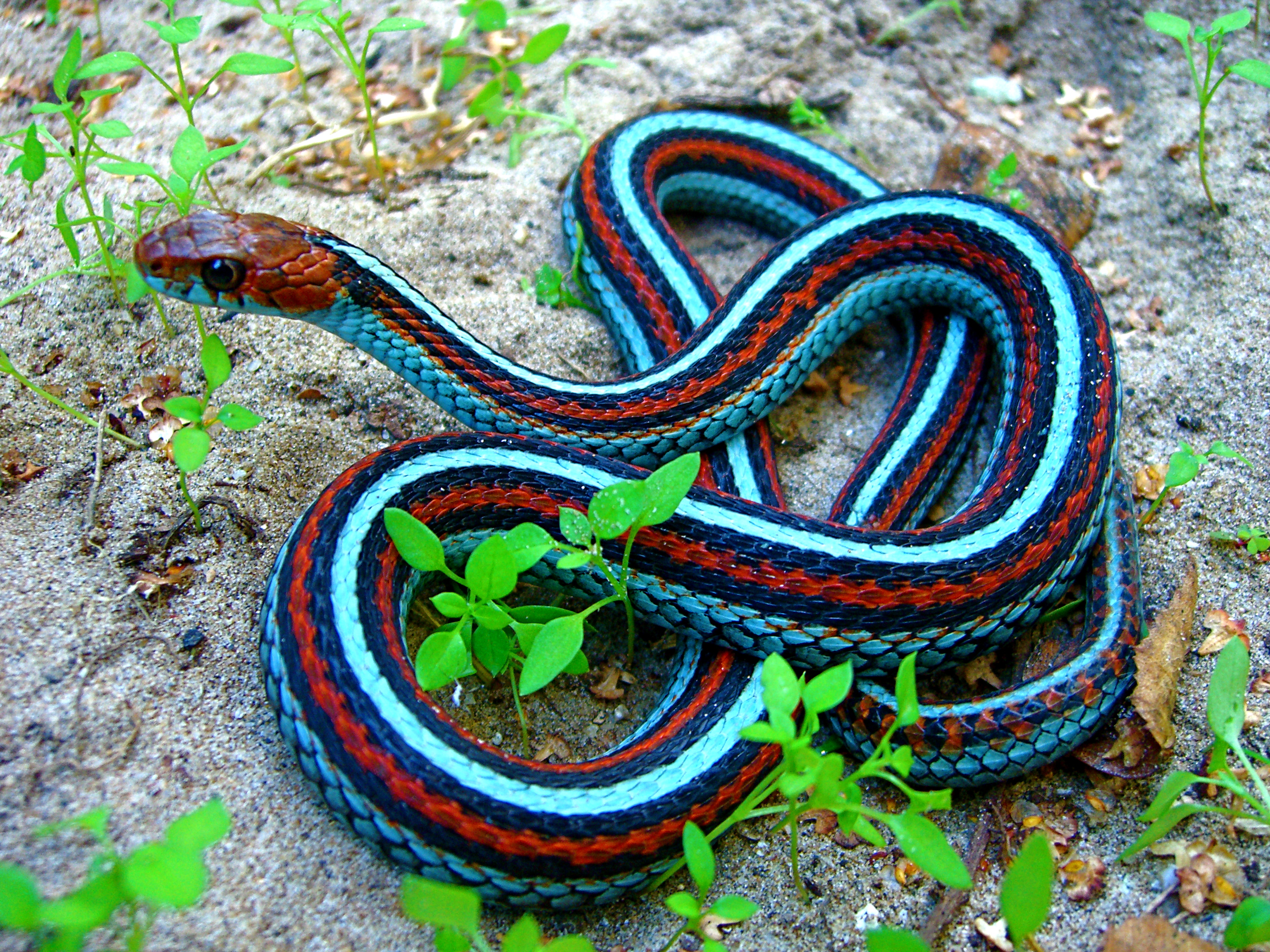The image features a striking snake, coiled gracefully on a grainy, light brown, beach-like substrate. The snake boasts vivid coloration with aqua and dark blue stripes contrasted by brownish-red bands, giving it an appearance reminiscent of a vibrant garden hose. Its head, directed towards the left, also displays the same brownish-red hue on top, while the underside is an eye-catching light blue. The snake's eyes are characterized by black centers encircled with brown. Surrounding the snake in the dirt are small, spindly green plants adorned with tiny teardrop-shaped leaves, adding touches of life to the scene. Scattered amongst the dirt are also a few dead, light brown leaves. While there is no text identifying the snake, it appears similar to garter snakes, which are commonly found in California according to some sources.